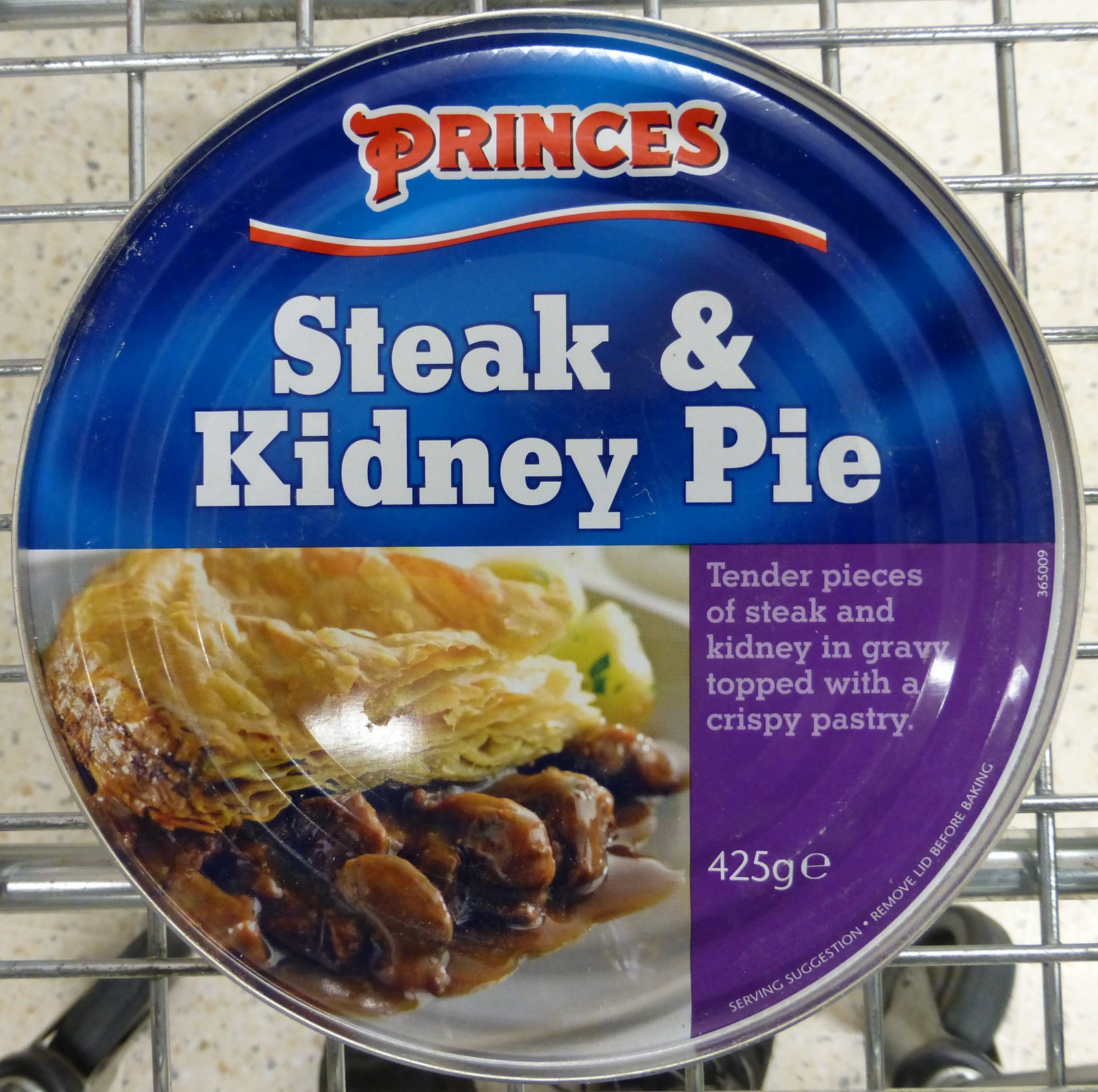This image is a detailed top-down photograph of a can of food placed in a shopping cart. The can prominently features a lid with the brand name "Princes" in bold red letters on a blue background, underlined by a white and red line. Below the brand name, in large white letters on the blue background, it reads "Steak and Kidney Pie." The lower section of the can's lid displays a color photo of the food, showing tender pieces of steak and kidney in gravy, topped with a flaky, crispy pastry. To the right of the image, within a smaller purple section, the description "Tender pieces of steak and kidney in gravy topped with a crispy pastry" is printed in a gray font. Additionally, a notation of "425G" with a symbol is visible in the purple area. The can itself sits on a chrome mesh, identifiable as part of a shopping cart due to the visible silver rods and a caster wheel in the corners of the image.